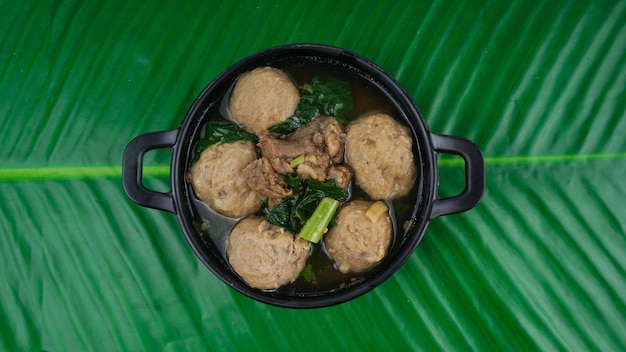This image features an overhead view of a matte black cast iron pot with two ring-shaped handles, sitting on a large, glossy green banana leaf with a light green stripe running through its center. Inside the pot, which is nearly filled to the brim with a darkish broth, float six meatballs, five of which are intact while the central one appears to be broken. In addition to the meatballs, the pot contains green leafy vegetables, likely spinach, along with visible chunks of carrot and onion. The liquid broth, just below the meatballs, provides a rich base to this substantial and inviting dish reminiscent of an Asian-style meatball soup.